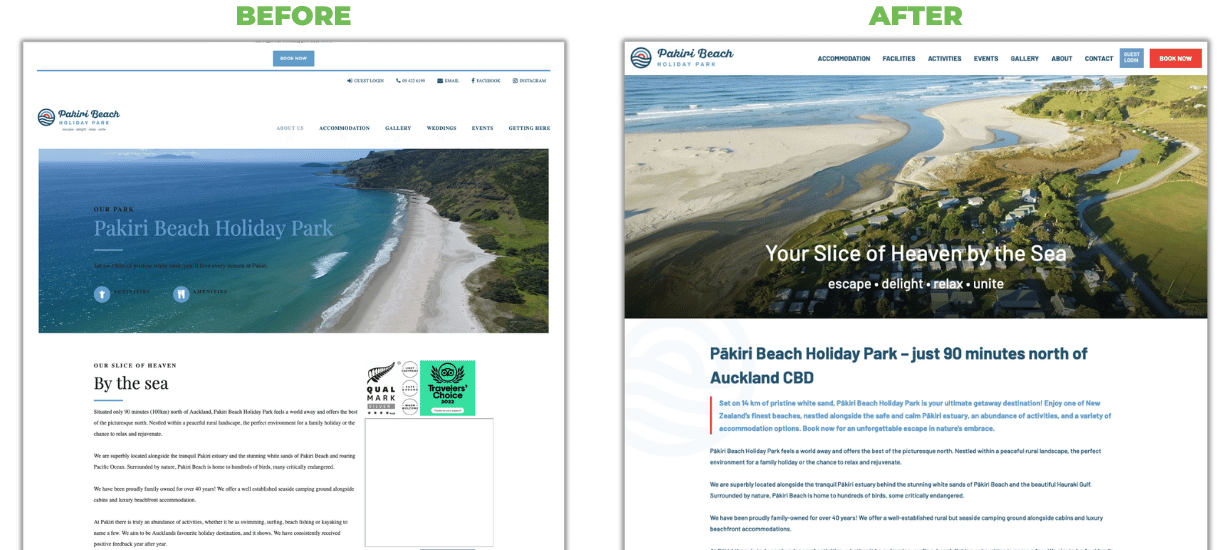### Before and After Screenshots of Pekere Beach Holiday Park Website Redesign

**Before (Screenshot 1):**
- The interface features a coastal theme with an image of the beach.
- The page is titled "Pekere Beach Holiday Park by the Sea," prominently displayed at the top.
- A white square box contains text elements including the words "Quah" and "Mark."
- A green square is also present, although its purpose is unclear.

**After (Screenshot 2):**
- The redesigned interface still prominently features the beach.
- "Pekere Beach" is the main header with several navigation items below it. These items include: Activities, Events, Gallery, About, Contact.
- A blue square is situated somewhere on the page.
- A red rectangular button labeled "Book Now" stands out for quick access to reservations.
- The image of the beach is accompanied by a view of some holiday homes further back.
- A slogan reads "Your slice of heaven by the sea. Escape, delight, relax, and unite," with the word "Relax" emphasized in bold.